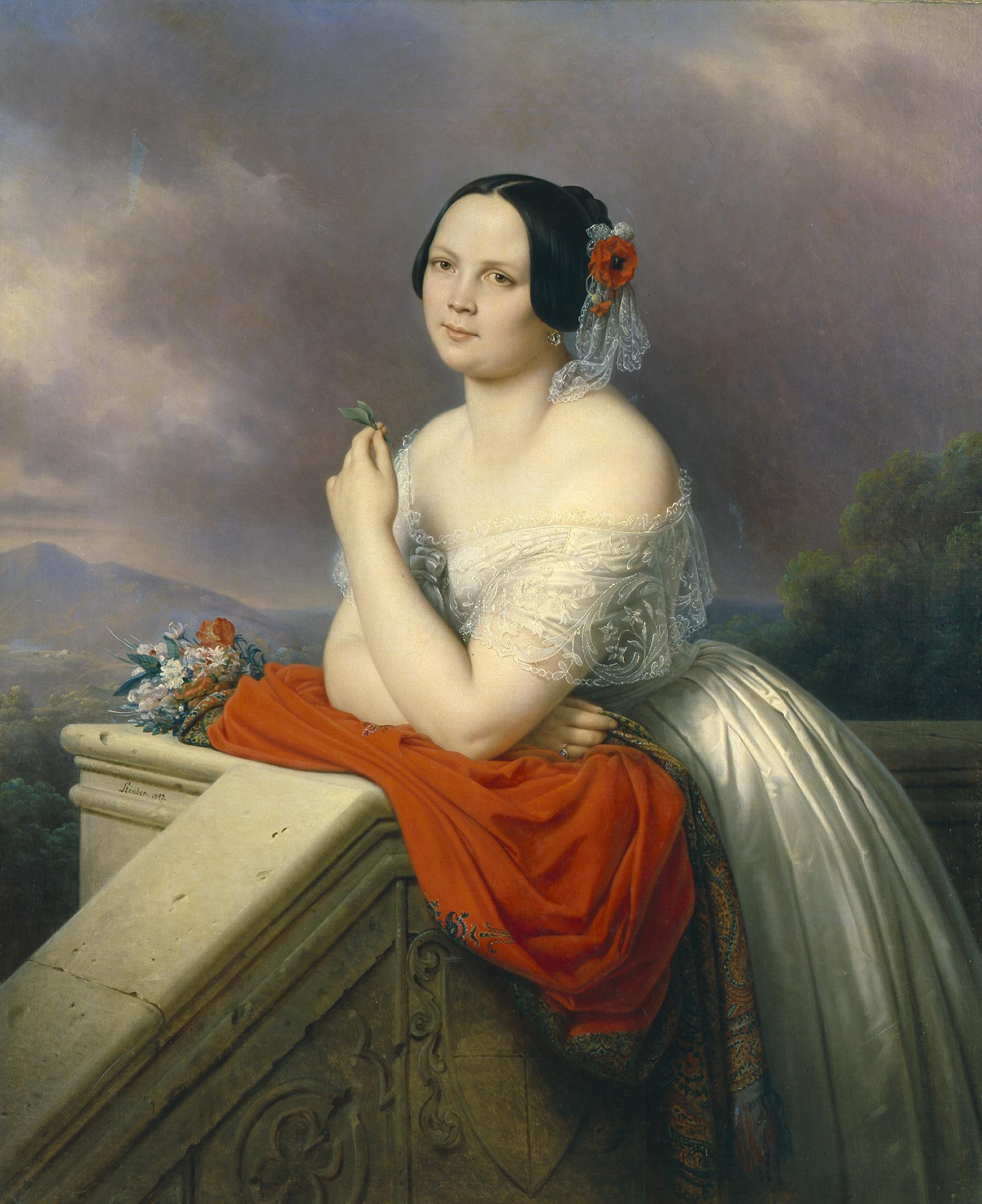This is a somber Renaissance-style painting portraying a Caucasian woman with dark eyes and black, shorter hair adorned with a white lace ornament and a red flower. She is wearing an off-the-shoulder gown made of white lace and silk, providing a striking contrast to her dark surroundings. The woman leans slightly over a half marble wall or staircase that features some inscriptions, with a red drapery or fabric gathered on the ledge. She is central to the image, gazing out towards the viewer.

In her hand, she holds a leaf, while her ring catches the light subtly. The background is evocative, featuring a stormy dark sky with heavy clouds, with hints of hills, bushes, trees with green leaves, and distant mountains, adding depth and atmosphere to the scene. The style suggests it might be a watercolor or oil painting, capturing a realistic depiction against the dramatic backdrop.